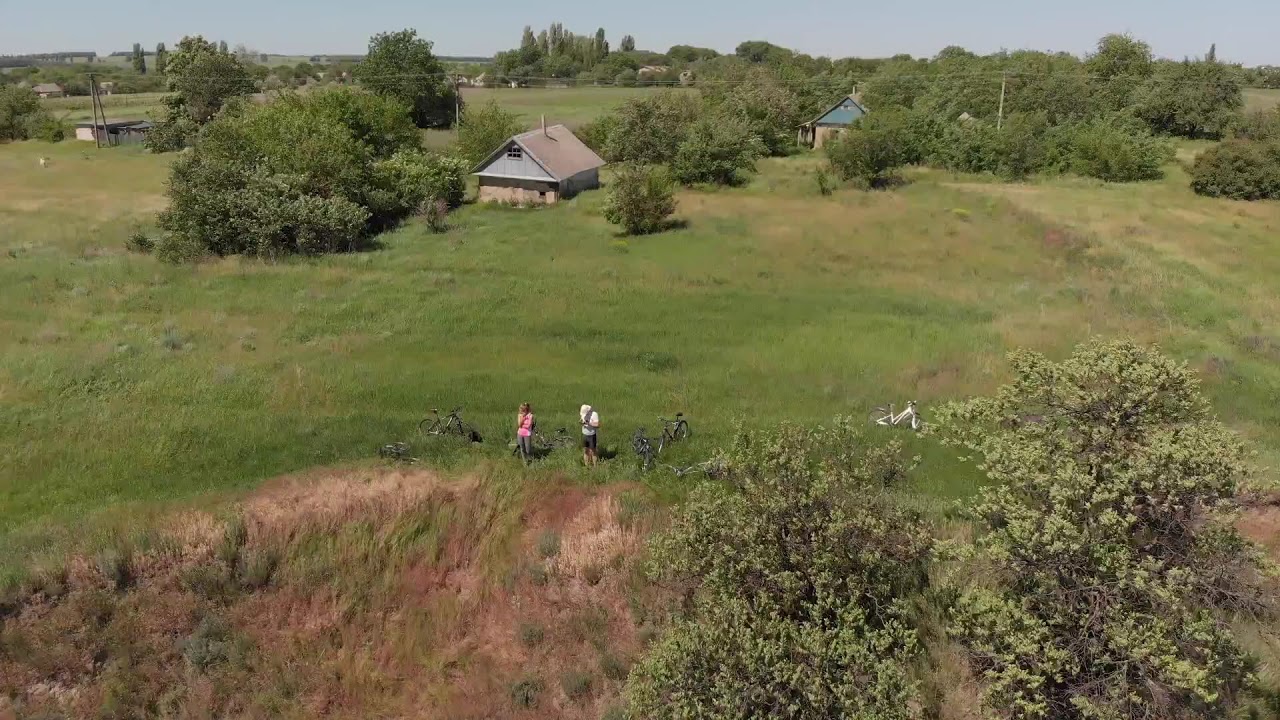The image presents an overhead view of a secluded, grassy field dotted with trees and sporadically placed houses. At the center, slightly to the left, stand two people with their bikes: one wearing a pink shirt with gray pants and the other in a white shirt with black biker pants; their three bikes—two black and one white—are arranged nearby. In the lower portion of the image, the terrain showcases a mixture of green brush and tan dirt, suggesting a hilly area filled with bushes and shorter trees. The homes, mostly tan, green, and occasionally blue or gray with triangular roofs, are scattered towards the top of the image, resembling an abandoned town devoid of connecting roads. Tall green trees line the background, with a hint of light blue sky or possibly a large body of water visible at the very top, further emphasizing the isolated, serene nature of this landscape.